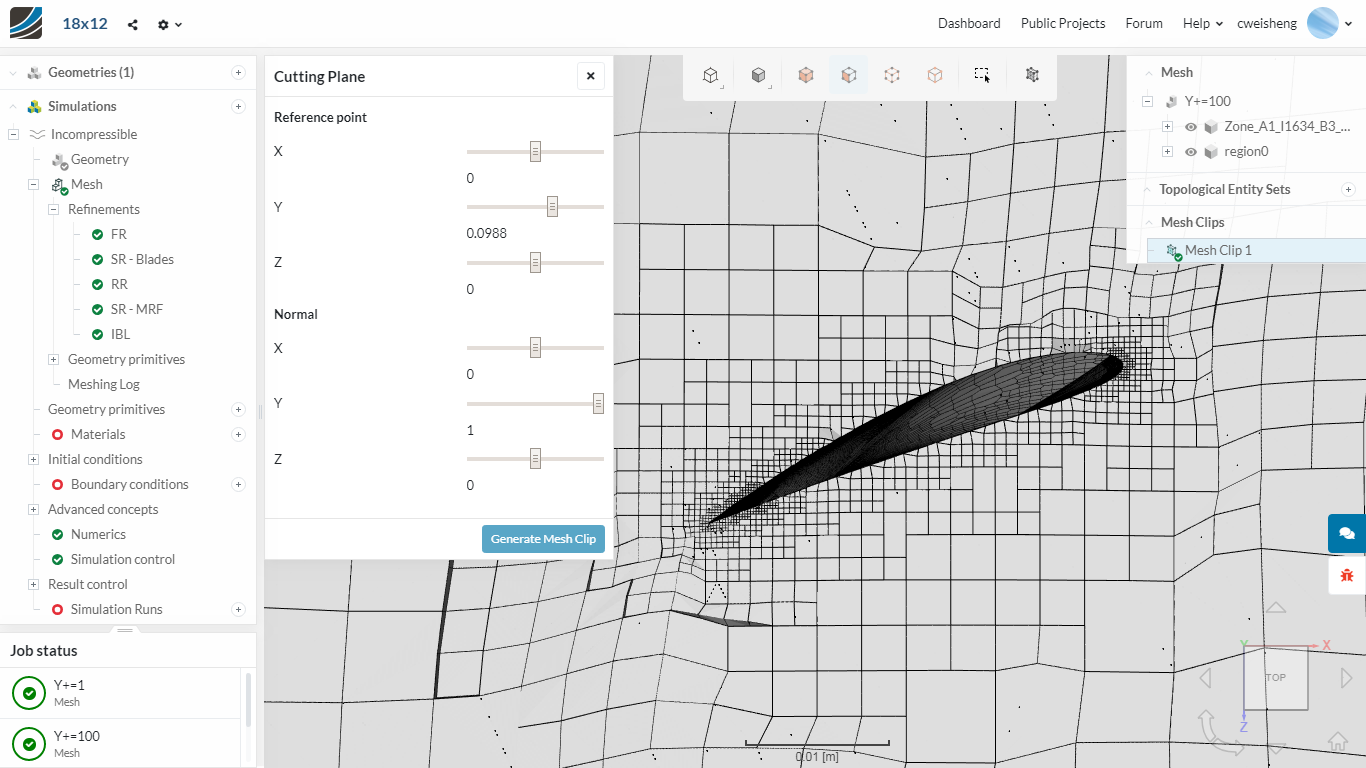The image is a detailed screen capture of a computer program displaying a complex map. The main visual is a horizontal rectangle with a predominantly gray background, intersected by numerous black lines forming a checkerboard pattern of squares varying in size, mainly concentrating in the top and lower right sections. Nestled within this map, an angled black oblong shape runs upward to the right. 

In the very upper left-hand corner of the screen, there's a small icon displaying blue and black stripes alongside the text "18 by 12". Next to this, there are gray labels such as "dashboard," "public projects," "forum," and "help", each of which are dropdown menus. The rightmost option in this series seemingly reads "Welshing."

To the left of the map, a vertical white rectangle titled "cutting plane" includes the coordinates x, y, z, accompanied by fields labeled "normal" and another set of x, y, z values, aligned downward. This section also features a blue button labeled "generate mesh clip."

Dominating the left side of the image is an extensive dropdown menu against a white background, listing options such as simulations, incompressible, geometry, mesh, refinements, and more, indicative of the program’s functionalities. The bottom of this menu displays the "job status" in black letters, accompanied by two green check-marked circles labeled "y plus equals 1" and "y plus equals 100", suggesting successful status tasks.